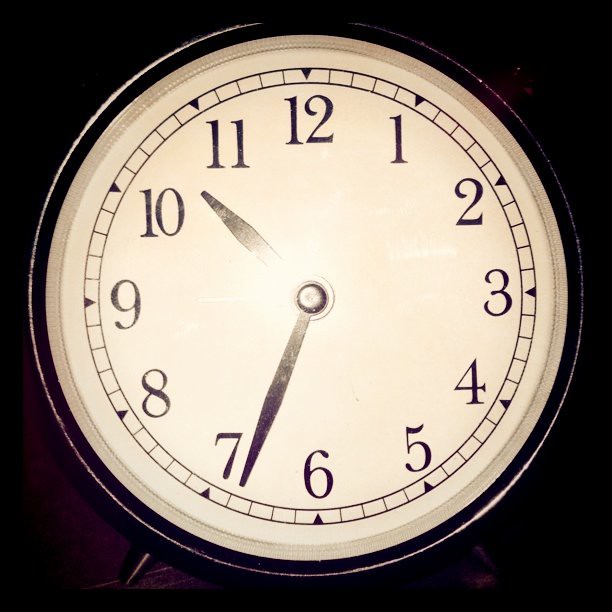This image portrays a desktop clock set against a black background. The clock features a white or off-white face encircled by a black frame, with black numerals ranging from 1 to 12 in a retro font. Surrounding the numbers is a series of rectangular minute ticks forming a circle, with bluish-purple reflective triangles pointing towards each numeral from inside their respective rectangles. The clock hands are black, showing a time of approximately 10:34, with the small hand positioned between 10 and 11, and the large hand located just past 7. While there is no second hand, one can observe what appears to be small legs on the bottom of the clock, suggesting that it is a desktop model.